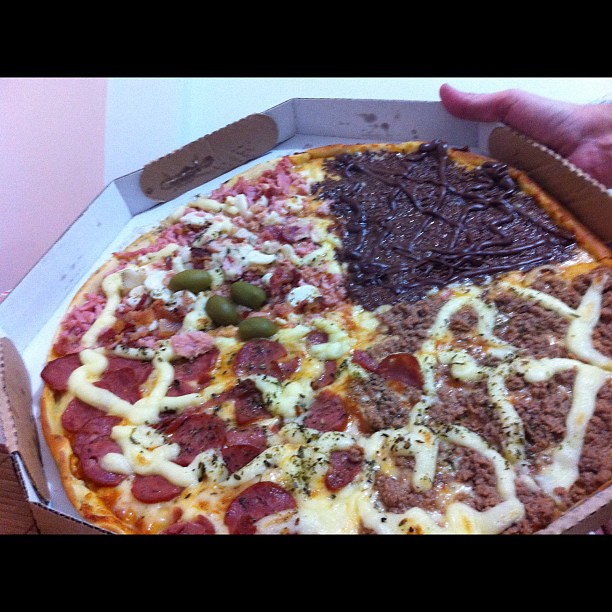The image shows a fully cooked pizza in an octagon-shaped, white to-go box, held by a hand with a visible thumb. The pizza is divided into four distinct quarters, each featuring different toppings. One quarter is topped with pepperoni, while another has Canadian bacon and olives. The third quarter appears to have chocolate and is further garnished with chocolate drizzle, resembling a dessert pizza. The final quarter contains hamburger or beef with a creamy drizzle that could be mayonnaise, crème fraîche, or ranch dressing. The crust is a golden brown, and the overall presentation suggests the pizza is ready for delivery or pickup.